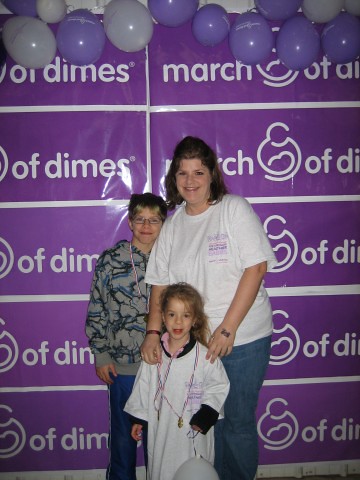In front of a repeating purple banner adorned with the March of Dimes logo, a group of three people stand closely together, likely family members. Above them, red and gray balloons add a festive touch. The central figure is a woman on the right, with dark black hair cascading to her shoulders and a radiant smile, revealing her teeth. She dons a white t-shirt with pink and purple writing on the chest area paired with blue jeans. In front of her stands a small child with strikingly bright red lips, wearing an oversized white t-shirt that drapes like a dress, with black fabric visible at the wrists. To the left, partially obscured by the woman, is an elderly lady wearing glasses. She has dark hair parted in the middle and is dressed in a gray, black, and blue-patterned top with blue jeans. The background, filled with purple squares, consistently displays the March of Dimes logo.